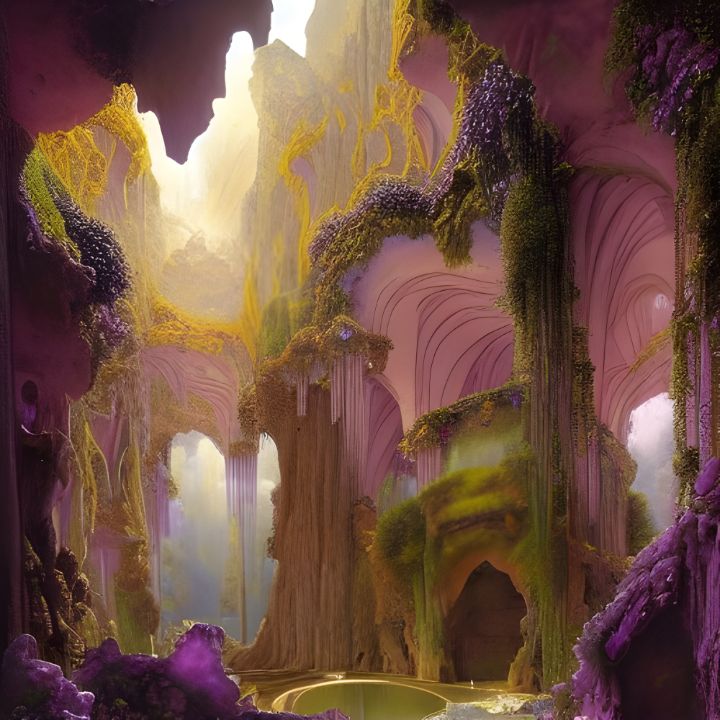The image presents an ethereal fantasy cave environment, suffused with lush, vivid hues of purple, pink, yellow, and green that render an otherworldly atmosphere. Light, both from above and potentially within the cave, casts a warm, ambient glow, filtering through and illuminating the interior with soft rays. The cave walls feature both smooth, curved surfaces and jagged, rocky textures. An abundance of moss and vine-like vegetation, some in a willow-like fashion, hang from the cave ceiling and walls, blending seamlessly with vibrant purple flowers.

A calm body of water or a reflective pond is situated at the cave's base, adding to the serene atmosphere. The presence of what appears to be a fireplace and archways suggest an architectural element, possibly evoking a setting reminiscent of "Lord of the Rings," with towering, canyon-like walls flanking either side and an archway in the center. The cave has multiple openings, some of which allow glimpses of the sky that beams light into the cavern, enhancing the dream-like quality. 

Crystallized rock formations in dark purple and lavender hues, along with a tapestry of plants, greenery, and dangling vines, add layers of detail and color. Towards the background, there's a doorway and paths leading outside, hinting at a labyrinthine expanse beyond. The whole scene is draped in fairy tale-like colors, blending deep purples, pinks, whites, and golds, suggesting both a natural and a slightly surreal, possibly AI-generated fantasy setting.